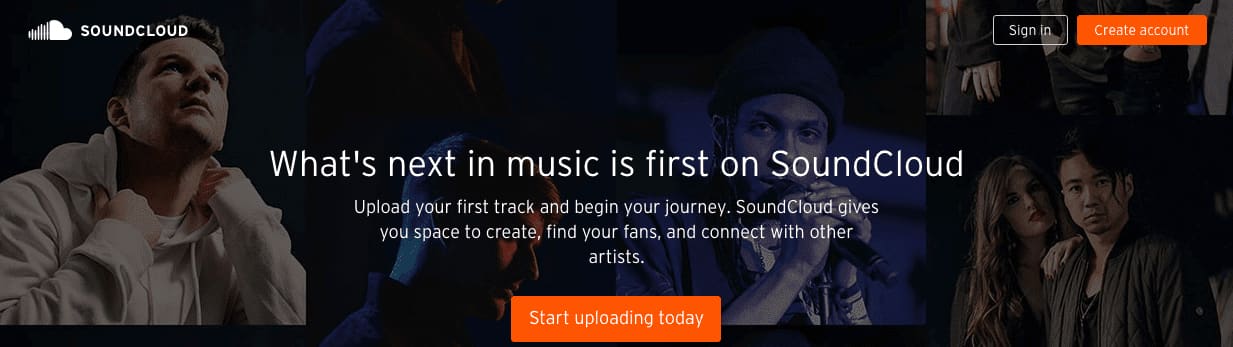In this image, the background is dark, contrasting sharply with a group of diverse individuals in the foreground. Among them, a young man in a white sweatshirt is looking straight up, while the others, who appear to come from different ethnic backgrounds, including one who seems to be of Indian descent and another of Asian descent, are looking more directly at the camera, each with a thoughtful expression.

In the upper left corner of the image, there is an illustration of a fluffy cloud with lines cutting through the left portion and a solid right portion. To the right of this cloud, "SoundCloud" is written in uppercase letters. Adjacent to this, there are two buttons: the one in a white box says "Sign in" in white text, while the one in an orange box reads "Create an account."

Center-aligned on the image is a captivating message in white text: "What's next in music is first on SoundCloud. Upload your first track and begin your journey. SoundCloud gives you space to create, find your fans, and connect with other artists." Below this message, there's a prominent orange button with white text that says "Start uploading today." The image is neatly designed and encapsulates the essence and the call to action for SoundCloud users.